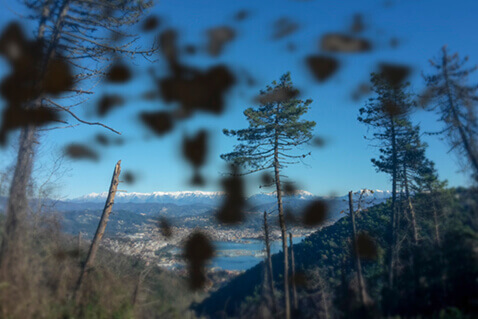The image captures a scenic landscape viewed from a higher elevation. The photograph reveals a forest scene with tall pine trees, their trunks mostly barren but crowned with green needles. Dirt spots, likely mud flecks, obscure parts of the image, especially on the upper left and center, indicating the camera lens was dirty. The scene unfolds with greener, shorter trees on a distant hill to the left side, descending towards a mid-ground valley, which harbors a serene blue lake. This lake with a slight inlet is encircled by greenery and the hint of a distant town. Beyond this tranquil setting, a majestic, snow-capped mountain range stretches from left to right, framing the backdrop. Above the mountains, a clear blue sky extends across the image, marred only by the smudges on the lens. The landscape illustrates a striking natural scene, capturing the harmony between the forest, the lake, and the looming mountains under an unblemished sky.